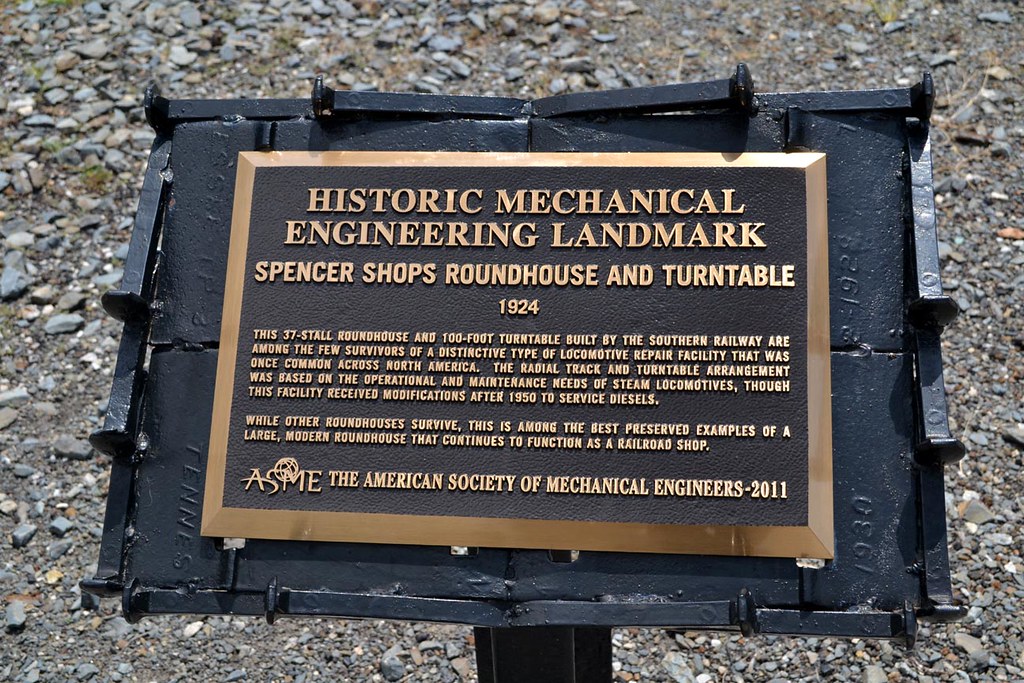The image depicts a wide rectangular outdoor sign on a black metallic surface framed by uneven nail-like objects resembling railroad spikes. The background features a gray gravel surface punctuated with occasional patches of grass. At the center of the frame is a gold plaque with a brown textured surface, inscribed in gold letters. The top of the sign reads "Historic Mechanical Engineering Landmark, Spencer Shops Roundhouse and Turntable 1924." Below, in smaller text, the plaque provides a detailed description: "This 37-stall roundhouse and 100-foot turntable built by the Southern Railway are among the few survivors of a distinctive type of locomotive repair facility that was once common across North America." It continues, mentioning that the roundhouse received modifications after 1950 to service diesel locomotives, and highlights its significance as one of the best-preserved examples of a large modern roundhouse that continues to function as a railroad shop. The plaque concludes with the text "The American Society of Mechanical Engineers, 2011."